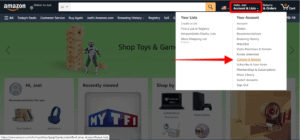A screenshot from the Amazon website displays various elements in a compact, rectangular format. At the top, the recognizable Amazon logo is featured in white with its signature orange smile beneath it. Directly below the logo is a white search bar encased in an orange outline, featuring a black magnifying glass icon. Next to the search bar, an American flag icon is visible, possibly indicating localization.

Highlighted in a red rectangular box is a section of white text, immediately followed by a white pop-up window containing black text. A prominent red arrow points towards a specific item under the 'Your Account' tab, which itself is highlighted in orange. Adjacent to this is the white Amazon cart icon.

A green advertisement banner resides at the top of the screen, promoting 'shop toys and games,' decorated with a Jenga tower graphic and a Power Rangers character set against a green background filled with black text. Below this ad, the 'Recently Viewed Items' section displays various items including a pair of blue headphones, several books, a Shopify filter category, a laptop, and what appears to be game systems. Despite the small size of the screenshot, the visual details remain clear and discernible.